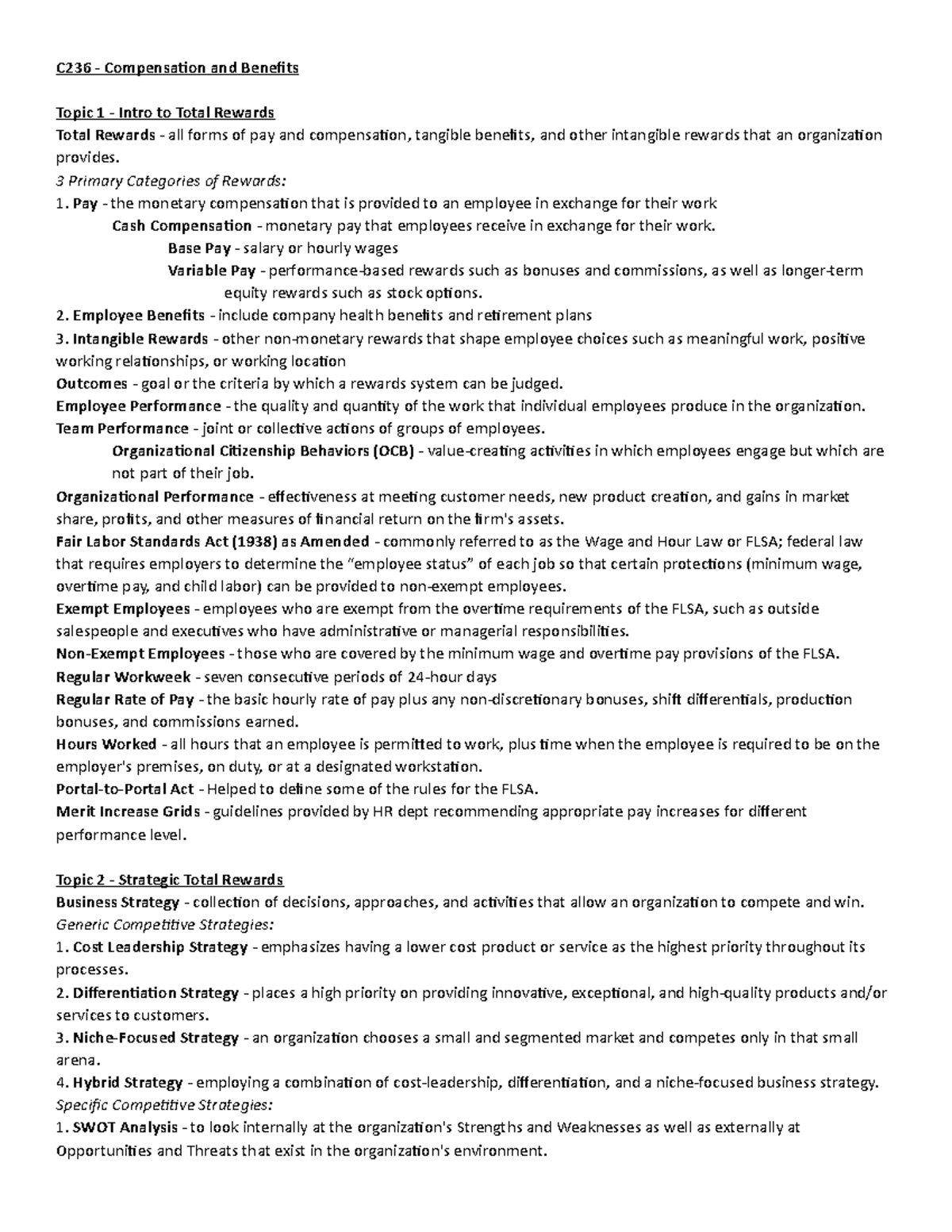The image depicts a printed sheet, either from a computer screen or a piece of paper, presenting a lengthy and detailed legal document. The document is titled "C236, Compensation and Benefits." It begins with "Topic 1: Intro to Total Rewards," explaining that Total Rewards encompass all forms of pay and compensation, tangible benefits, and other intangible rewards that an organization offers. The section further categorizes rewards into three primary groups: Pay, Employee Benefits, and Intangible Rewards, each of which is defined in detail. Moving on, "Topic 2: Strategic Total Rewards" is introduced, listing four strategic approaches: Cost Leadership Strategy, Differentiation Strategy, Niche Focus Strategy, and Hybrid Strategy, all accompanied by their respective definitions. This page clearly represents just one segment of what appears to be a significantly extensive document.